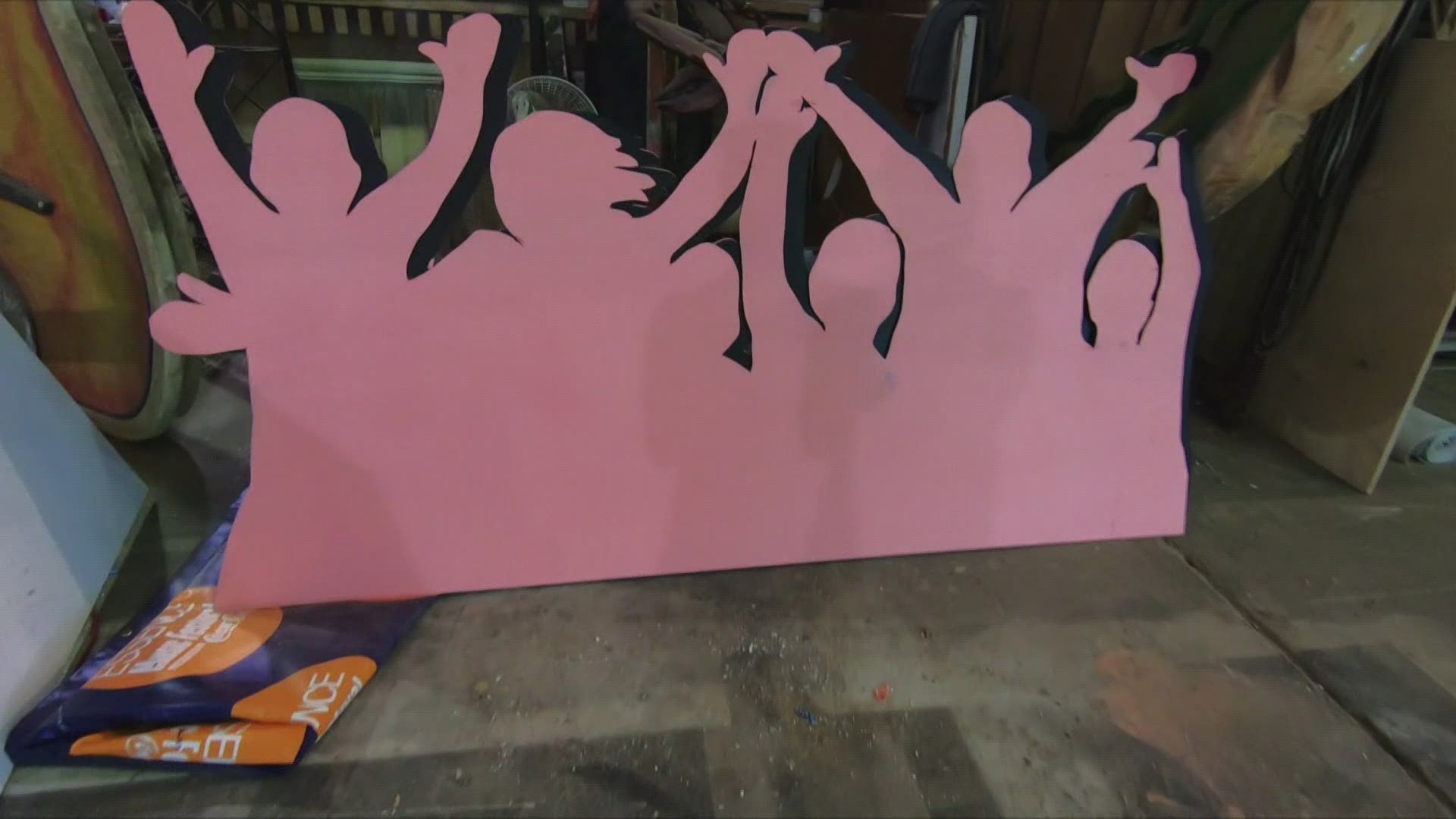The photograph, taken in a landscape orientation, depicts a vibrant and detailed indoor scene within a workshop. The primary subject of the image is a large pink silhouette made from cardboard or poster board, depicting a diverse group of people enthusiastically raising their hands in the air. This cutout features six figures, including what appear to be two adults on the left and right sides and three or four children in between. The silhouette stands against a gray wall with various shadows cast over it, indicating the presence of the photographer or someone else in the room. On the left side of the cutout, there’s a folded blue and orange paper bag.

The room's floor is made of wood planks, which are either laminate or hardwood, and is clearly used for creative or production purposes as it is marked with paint splatters. This adds to the impression that the space is utilized for constructing props or art pieces, possibly for a play or musical performance. In the background, there is a table with visible wooden legs and other workshop materials scattered around, adding layers of context to the setting. The overall scene is bathed in a natural realism, capturing the essence of an active, artistic workspace.